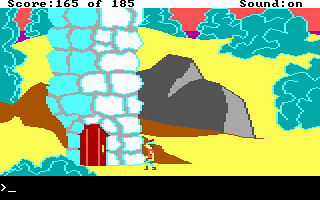This is a highly detailed, computer-generated image depicting a scene from a video game. At the top of the image, game elements are displayed, including a score of 165/85 and an indication that the sound is on. The focal point is a majestic stone castle featuring a prominent tower. The stones are distinctly outlined with plaster, revealing meticulous construction details. The tower's stones are colorfully divided; the lower half showcases a light blue hue, while the upper half transitions into a pristine white. Adding a touch of realism, the castle tower includes a sturdy brown door framed by an arch composed of alternating light blue and white stones. In the background, whimsical bluish bushes contrast against large, dark stones, creating a fantastical environment. Positioned in the foreground is a character poised to run, ready to embark on the next adventure in this captivating game world.